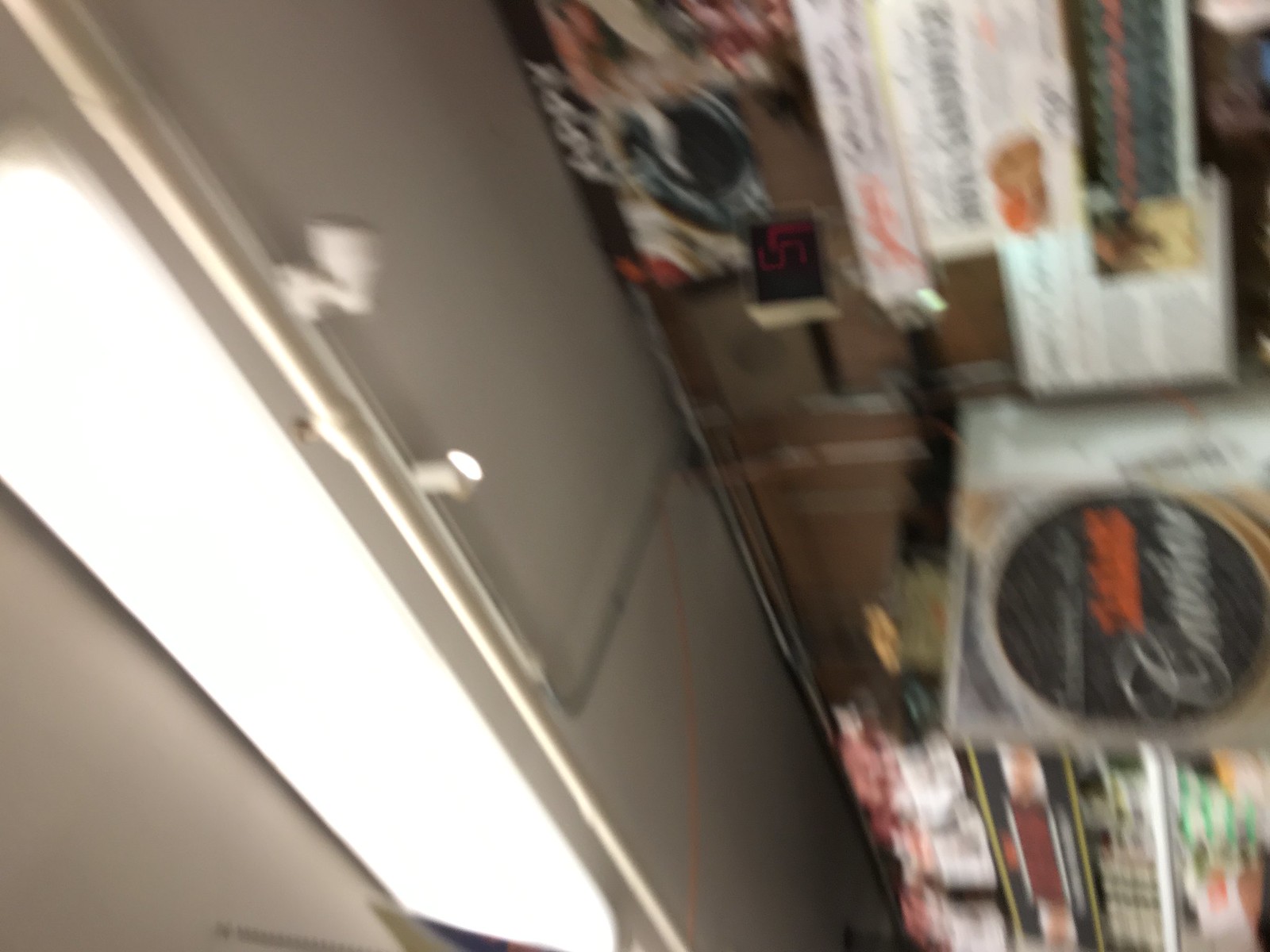This is a blurry, color photograph taken at a sideways angle, possibly depicting the roof of a shop or an interior setting like a store or a room. The main feature is a white object resembling a refrigerator or square pillar, with poles extending from it, possibly supporting track lighting. The roof or ceiling features both white and tan colors, with white track lighting fixtures. The background includes a variety of colorful items, possibly small appliances or store products like cigarettes, displayed on shelves or racks. There are various colors visible, including red, black, green, orange, and white, though the exact items and writing are indistinguishable due to the blur. Additionally, there is a small board with a black circle containing writings in white and orange. The overall space appears crowded or compact. The image's angle further adds to the challenge of clearly identifying the objects within it.